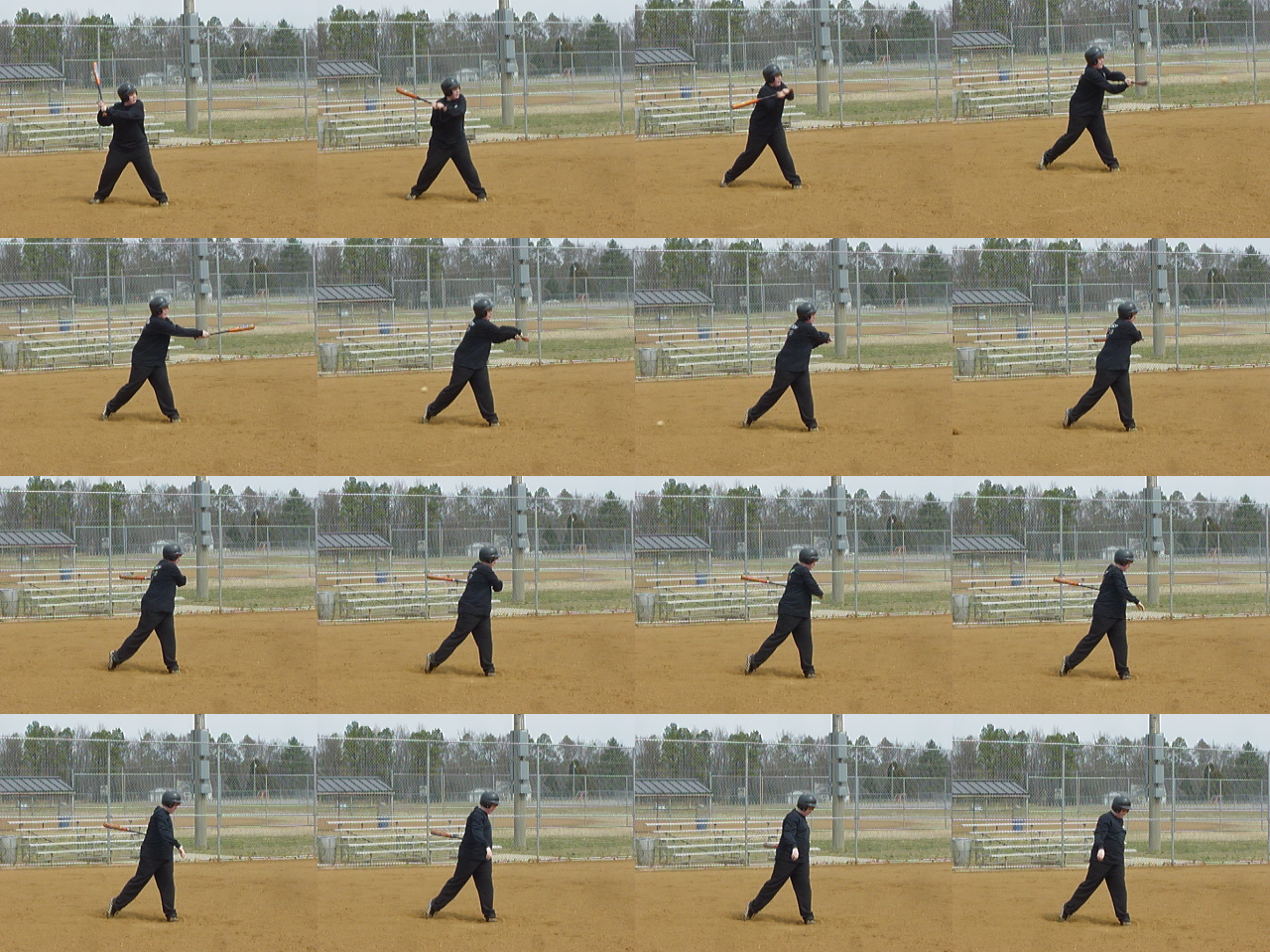This image is a composite of 16 still frames capturing the various stages of a young baseball player at bat, organized in four rows and four columns. Each frame sequentially documents the boy in a black tracksuit, black jogger pants, black long-sleeved sweatshirt, and black batter's helmet swinging an orange and black bat. The sequence progresses from the initial batting stance in the top left frame to the final follow-through in the bottom right frame. Throughout the images, the bat appears and disappears as it moves behind him during the swing. The boy is positioned on a dirt area, indicative of a baseball diamond, with bleachers, a chain-link fence, and trees visible in the sunlit background, suggesting a sunny day at a park. Notably, the ball itself isn't visible in any of the frames, giving an impression of hitting an "invisible ball."